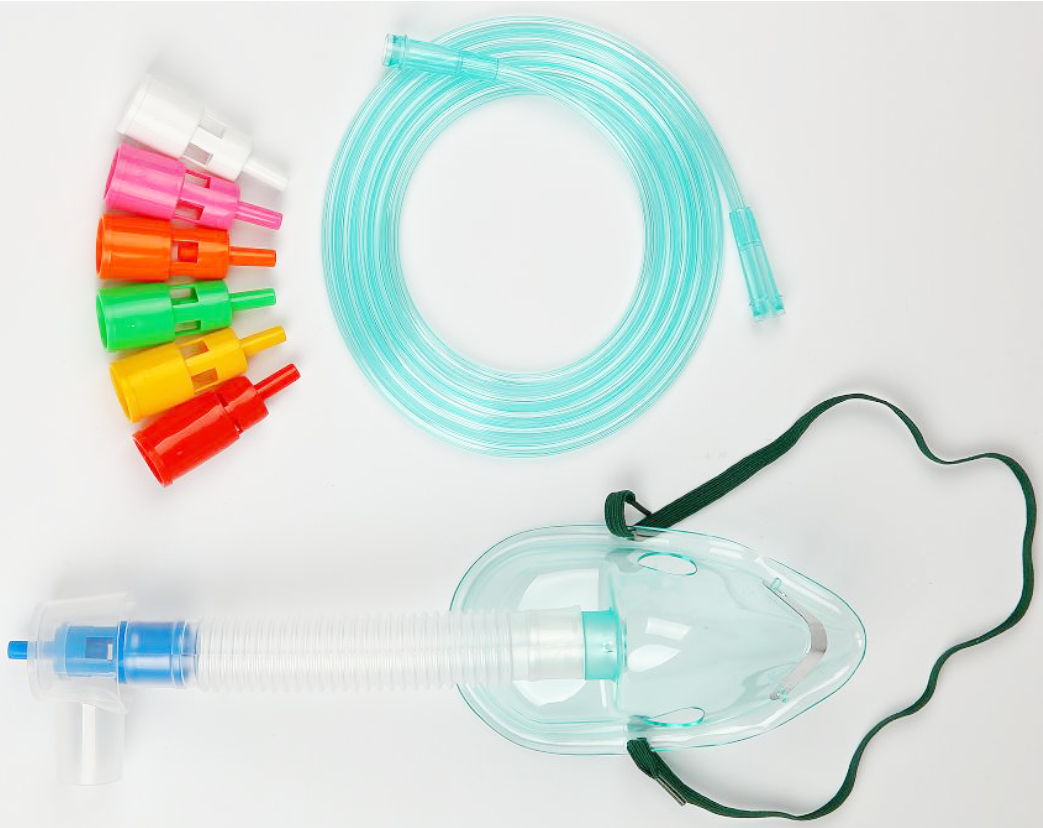This detailed photo captures a top-down view of medical equipment, specifically showcasing a ventilator mask setup. At the bottom of the image, there's a light green, transparent oxygen mask equipped with a dark green elastic strap that resembles a shoelace, attached to both sides. The mask features a transparent tube connected to its front, ending in a blue valve to the left. Centrally positioned above the mask is a coiled light green tube. To the left of this tube, there is a series of color-coded, hard plastic valves arranged vertically from top to bottom in white, pink, orange, green, yellow, and red. Each valve appears to have different sized holes, potentially for controlling the airflow. The entire setup is organized on a white platform, providing a clear view of the components.